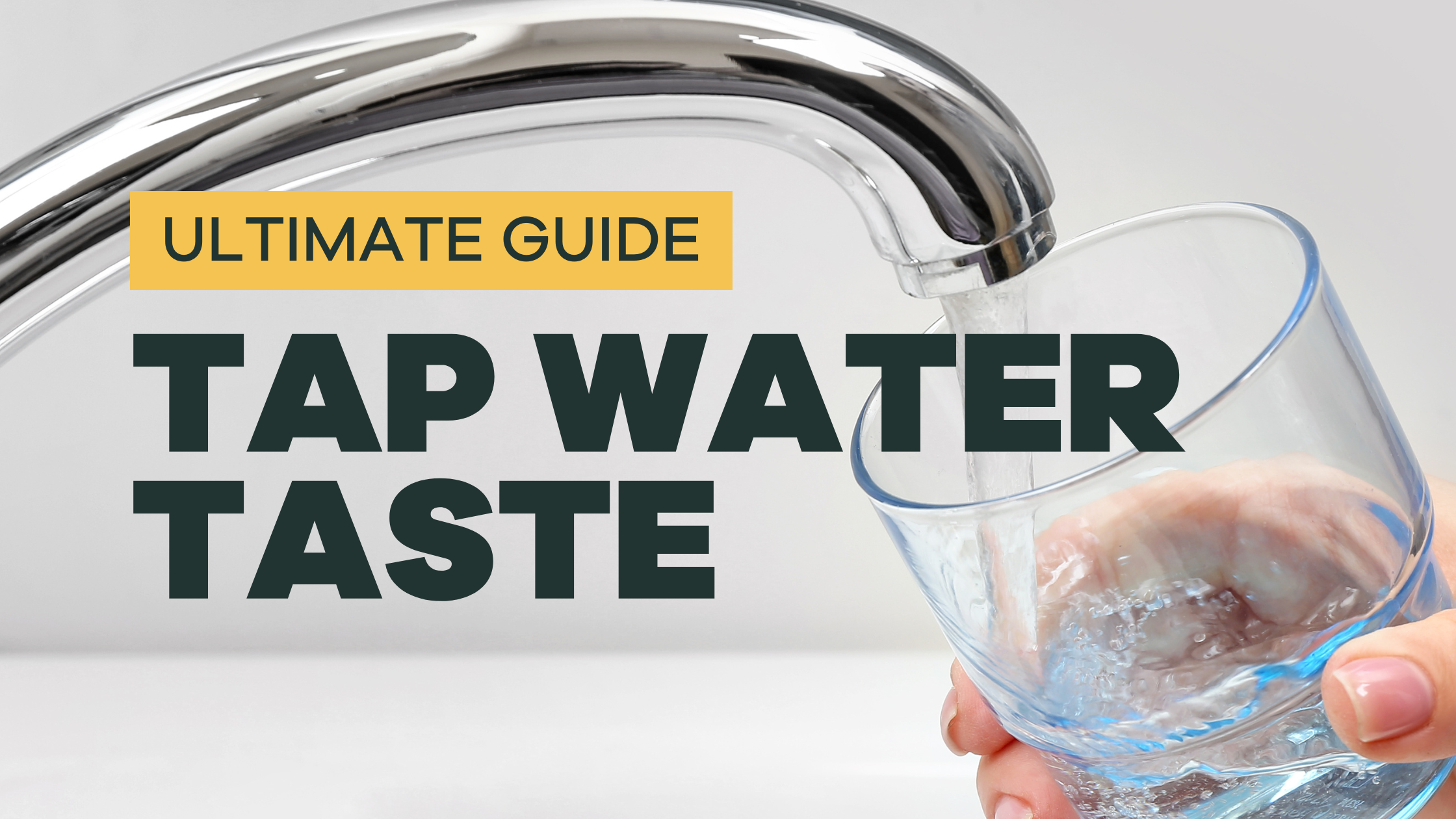This image is an advertisement or informational booklet with a very bright background predominantly featuring a sleek, shiny silver faucet in the upper left corner, pouring water. The backdrop is a plain white wall, emphasizing the vibrant elements in the foreground. At the top of the image, a yellow banner reads "ULTIMATE GUIDE" in black lettering, beneath which are large, all-caps letters spelling out "TAP WATER TASTE." 

In the lower right corner, a female hand with well-manicured, clear-lacquered nails is holding a small, heavy-bottomed glass, around four to six ounces in size. The glass, partially filled with water, has an enhanced blue tint, creating a vivid contrast with the clear stream of water pouring from the faucet. The overall composition is simplistic yet visually striking, with a clear focus on the act of filling a glass with tap water.